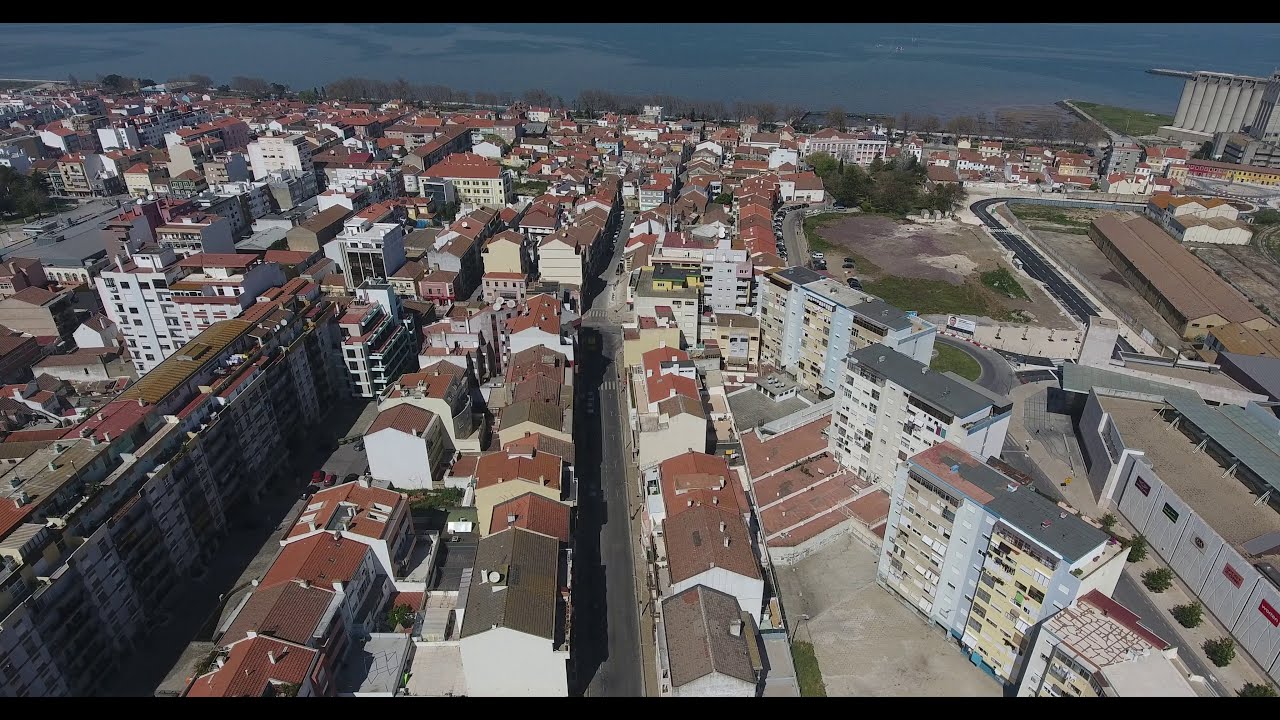This detailed aerial photograph showcases a densely populated town or city situated beside a large waterway, likely a river or lake given the absence of waves. Captured in landscape horizontal format by a drone or airplane, the image reveals a meticulously organized residential area with streets running vertically from the foreground to the background. The rooftops in the foreground, mostly peaked and colored in clay red or dark gray, align neatly along these streets, getting smaller as they extend toward the background.

The town is predominantly composed of residential buildings with light-colored exteriors, mainly white, off-white, or yellow. The streets are interspersed with regular intervals of roads, some dotted with moving vehicles, indicating a bustling community. Towards the far end, a striking blue waterway stretches from the left to the right edge of the image, marking the boundary of the town.

In the lower-right corner of the photograph, three high-rise apartment buildings standing seven or eight stories tall can be observed, distinguished by their flat gray roofs and white facades with balconies. These buildings are slightly tilted at a 30-degree angle, adding a unique perspective to the uniform rows of houses. This area, likely a commercial district, contrasts with the residential zone due to the presence of several one-story commercial buildings with wide structures and large parking lots, suggesting storage units or similar facilities.

Despite the overall lack of green spaces, the background also hints at treetops near the waterway, adding a touch of nature to this highly urbanized setting. The clear daylight and sunlight falling on the surroundings firmly place the photograph in the daytime, capturing the vibrant essence of this meticulously structured seaside town.